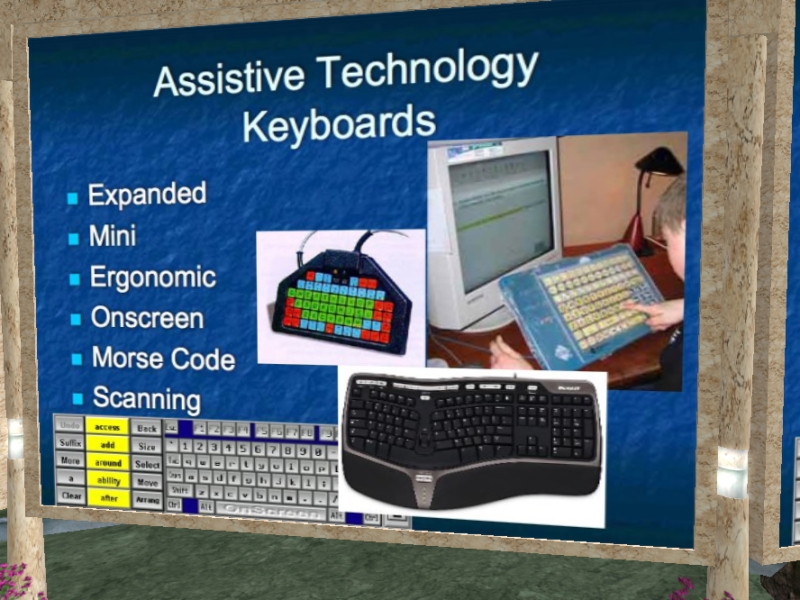The digitally created landscape-format poster, framed with a wooden effect, features white text on a textured dark blue background that reads "Assistive Technology Keyboards" across the top. Running down the left-hand side are blue square bullet points with white text listing various types of keyboards: Expanded, Mini, Ergonomic, On-Screen, Morse Code, and Scanning. The bottom left corner of the poster shows an image of a standard black keyboard, partially overlapping another keyboard in the top right of the first, both depicting different ergonomic designs. On the right middle side of the poster, there's a real photograph of a child interacting with a blue keyboard connected to an older CRT computer monitor, capturing a side partial silhouette. Additionally, there is an image of a keyboard with colorful red, blue, and green keys placed to the right of the bullet points. Below the poster, artificial grass is visible, adding to the digitally composed appearance of the presentation.